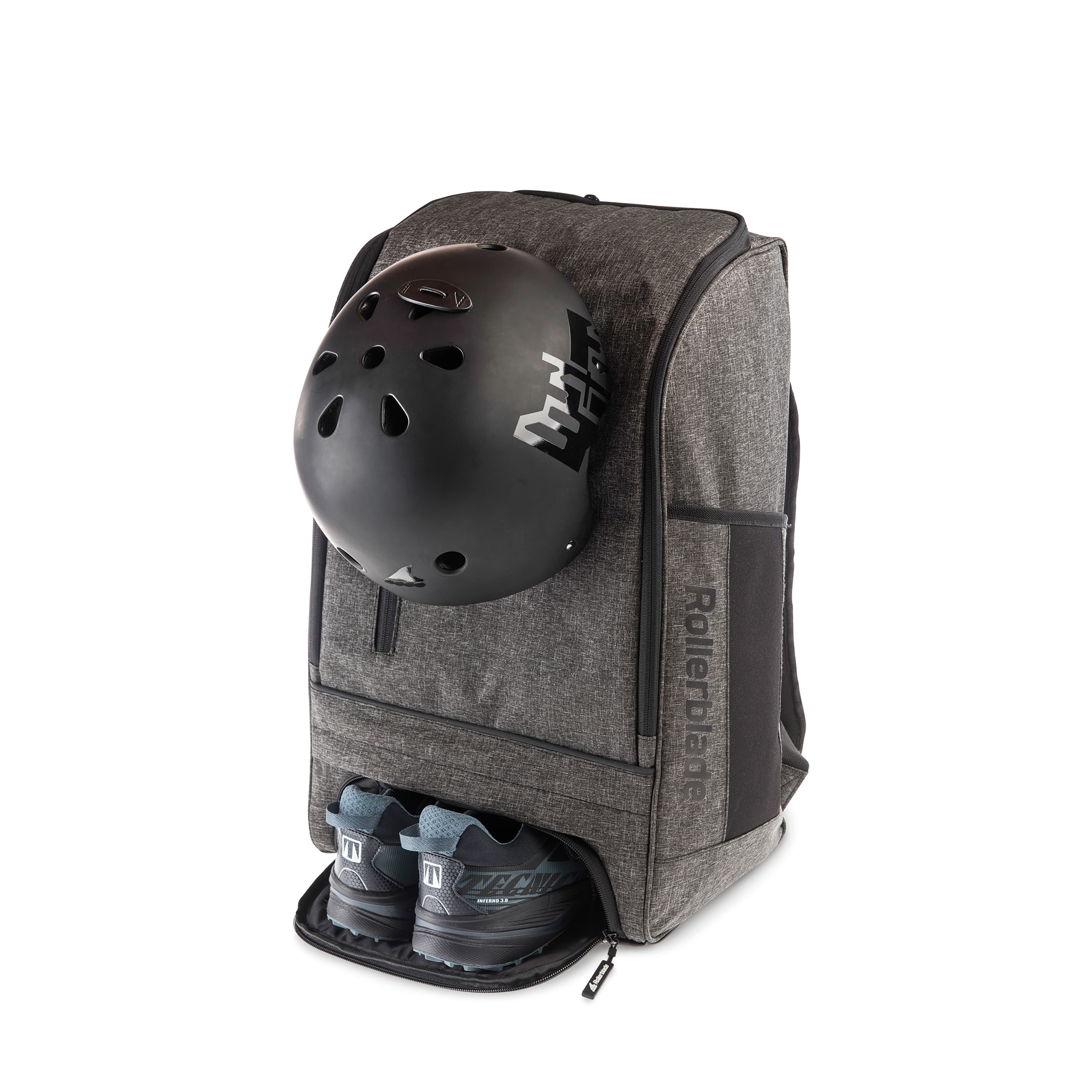This color photograph, presented in a portrait orientation, showcases a sleek, gray tweed backpack designed specifically for extreme sports enthusiasts and rollerbladers. The backpack features black accents and multiple zippers, including a prominent double zipper that starts at the top and goes all the way around the sides, enabling the main flap to fully open. There is an attachment on the back to hold a black helmet, which hangs down from the left side and features shiny graphics and ventilation holes on it. The right side of the bag has a black pocket, prominently displaying the word "Rollerblade."

At the bottom of the backpack, an unzipped compartment reveals a convenient storage space for shoes, lined with a protective rubber mat to prevent wet shoes from damaging the bag's contents. Two gray tennis shoes, with their heels facing outward, are partially stowed in this compartment. The bag also includes a small zipper on the back, ideal for securing small items like a wallet. The entire product is photographed against a clean, white background, emphasizing its features and giving it an advertisement-like appeal.